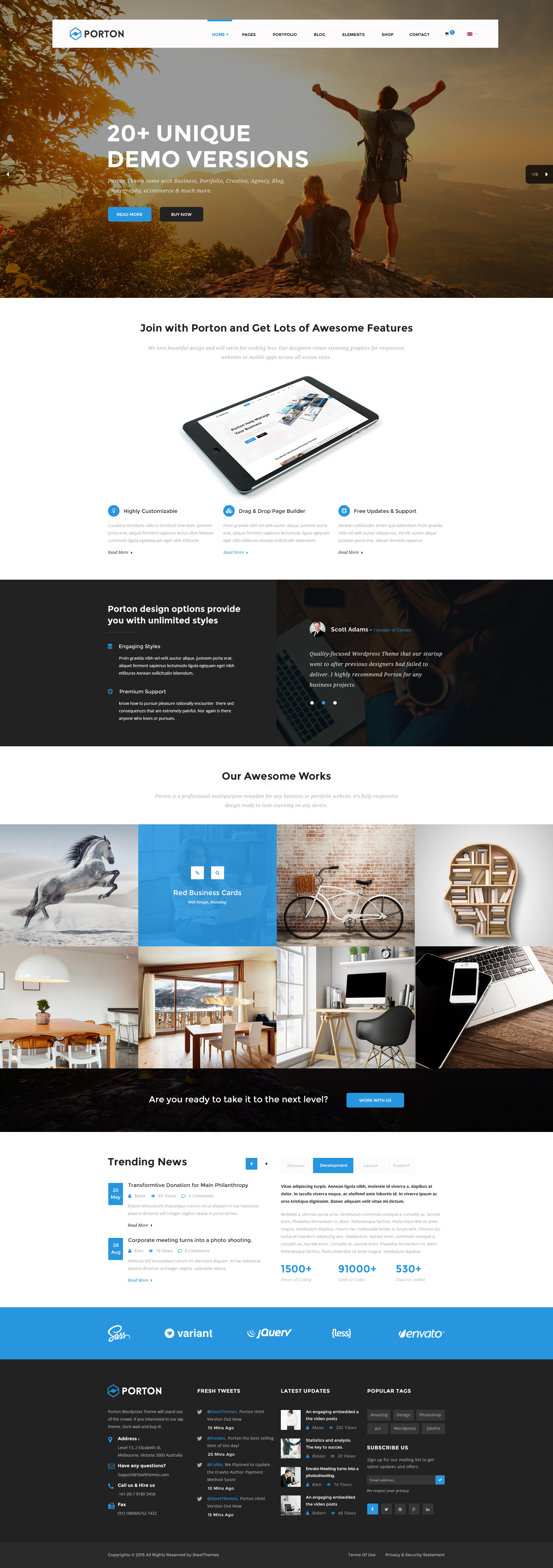This image displays a sophisticated web page layout for Porton, showcasing various categories and features designed to cater to multiple needs. The navigation bar includes links to Home, Pages, Portfolio, Blog, Elements, Shop, Contacts, and Cards. Highlighted features include "20+ Unique Demo Versions" and the extensive customization options available with the Porton theme, which supports Business, Portfolio, Creative, Agency, Blog, Photography, E-Commerce, and more. Prominent call-to-action buttons invite users to "Read more," "Buy now," and "Join with Porton to access numerous awesome features." A section for Trending News headlines current topics like "Transformative Donation from Main Philanthropy" and "Corporate Meeting Turned Into Photo Shooting." The overall message encourages viewers to elevate their website experience by partnering with Porton, asking, "Are you ready to take it to the next level? Walk with us."